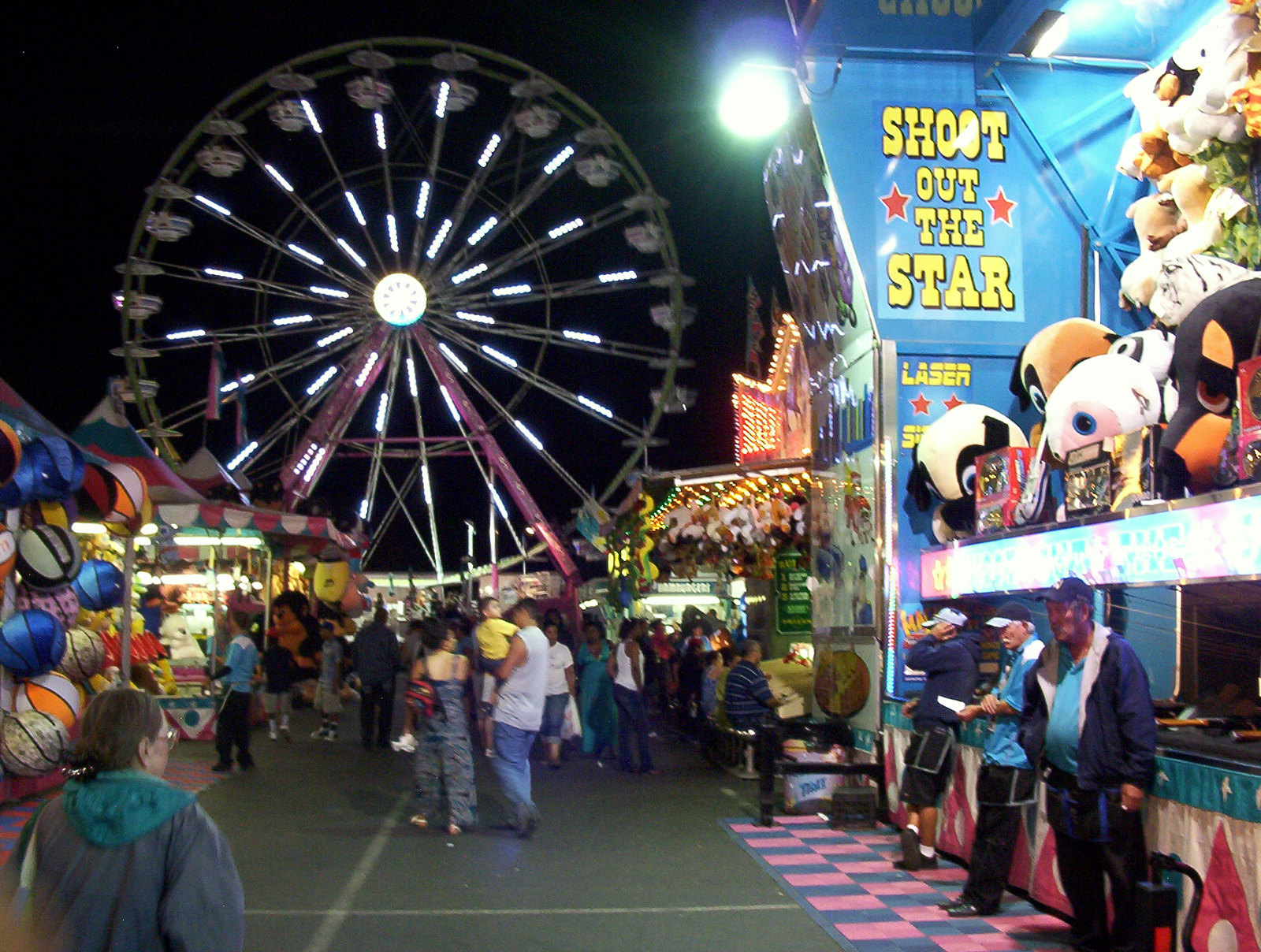This outdoor night-time festival or carnival scene is captured in a large, slightly blurry square photograph. Dominating the image, a Ferris wheel on the upper left is vividly illuminated with white lights against a solid black sky. Below, a variety of colorful canopy tents in blue, red, and white can be seen. To the far left, there's a row of basketballs displayed. The image's focus shifts toward the crowded middle ground, where a man in a sleeveless white shirt and jeans is carrying a little boy dressed in a yellow shirt. Nearby, a woman with glasses and brown hair, clad in a gray and green hooded jacket, is seen from the back.

On the right side of the image, multiple game stands are visible. A prominent blue wall labeled "Shoot Out the Star" in yellow letters, flanked by red stars, stands out. Above this game, numerous stuffed animals are lined up on a shelf. Three men, possibly vendors, are positioned in front of this game; two wearing blue jackets over light blue shirts, with different combinations of black slacks and shorts. The atmosphere is one of vibrant activity and leisure, with other people strolling down the center pavement, including couples and groups, enhancing the essence of a bustling fairground.